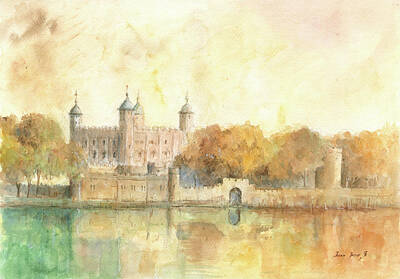The image depicts a vibrant painting—possibly watercolor, digitized, or oil-based—featuring a grand medieval castle with a striking array of spires topping its multiple towers. The castle, seemingly composed of sandstone, exudes an impressionistic and golden sunshine glow, with noticeable hues of brown and gray. The structure is set against a richly colored sky, blending shades of yellow, light brown, pink, and orange, which reflect onto the serene body of water in the foreground. Lush trees with a spectrum of green, orange, and yellow foliage flank both sides of the castle, enhancing the scene's natural beauty. At the bottom right, there's an artist's signature, rendered in a three-part squiggle, although too small to discern clearly. The composition cleverly uses reflective techniques to mirror the sky's colorful palette on the water's surface, encapsulating a warm, light-filled atmosphere.